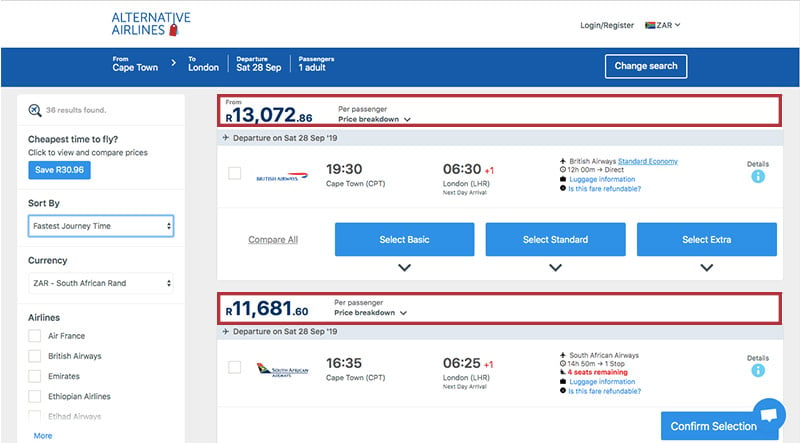The image is a screenshot from the web page of "Alternative Airlines." Displayed prominently at the top is a blue rectangular banner. Below this are various flight ticket options in red and blue, each representing different fare categories. 

To the right, a pricing column lists detailed fares, including a highlighted price of $13,072.86 per passenger, which might be calculated using points. Another notable fare is $11,681.60, enclosed within a long, skinny red rectangle.

Beneath the fare options, there are sections labeled "Select Basic," "Select Standard," and "Select Extra" within blue boxes. The bottom right-hand corner features a blue box with the text "Confirm Selection."